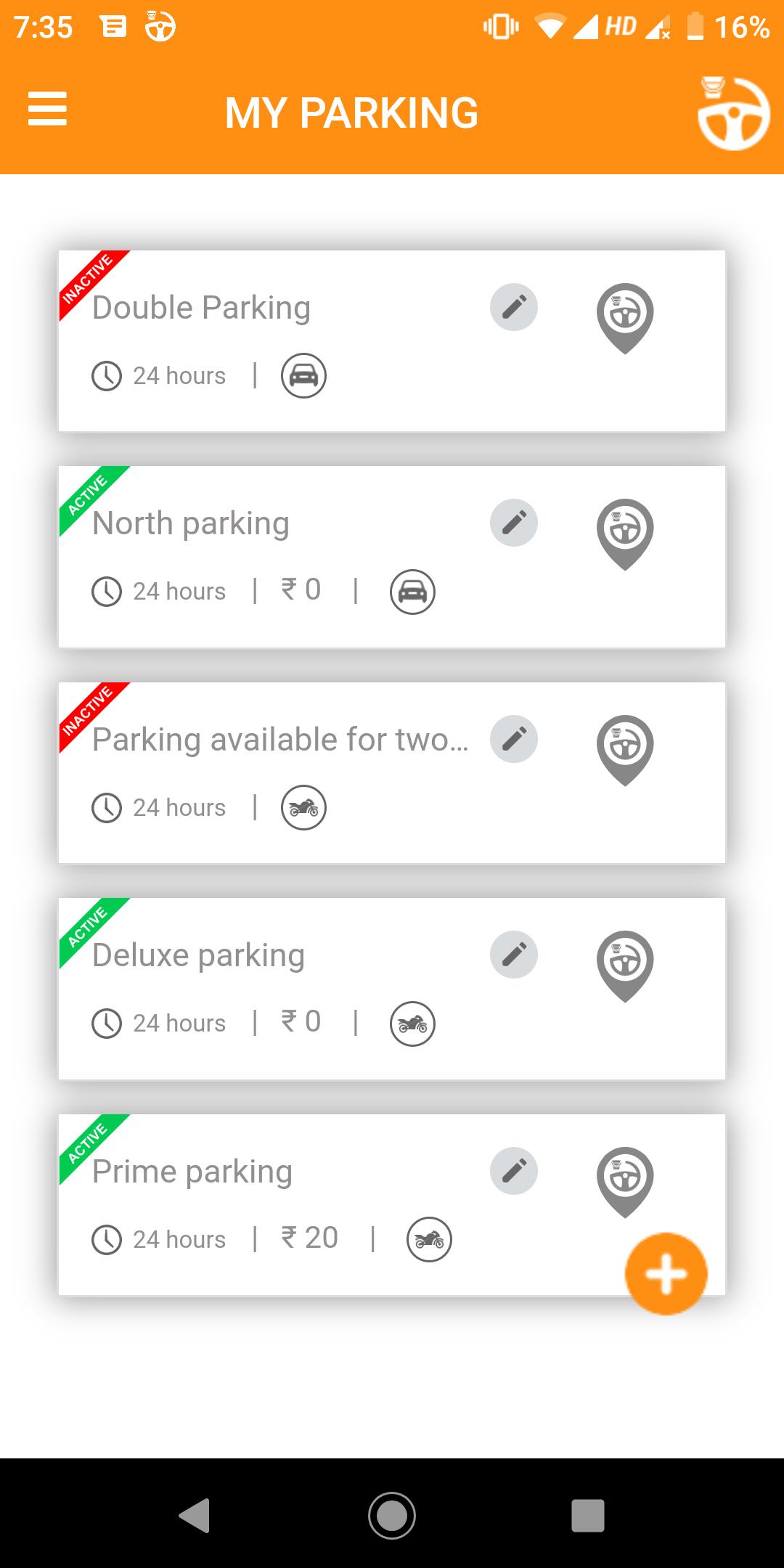Screenshot of a Cell Phone Displaying Parking Locations:

The image is a screenshot captured on a cell phone, featuring details related to various parking locations. The interface has an orange border at the top. At the top left corner, the time displayed is 7:35. To the right of the time are several icons: a notes icon, a steering wheel icon, a phone vibration icon, Wi-Fi signal, cell signal strength, "HD" indicating high-definition voice capabilities, and a battery indicator showing a 16% charge. 

Centered within the orange border, in white text, is the title "My Parking." On the far right side of the orange border is a white steering wheel icon with a small car symbol in the upper left-hand corner of the steering wheel.

The main portion of the screenshot has a white background featuring five horizontally aligned rectangular boxes, each providing details about different parking spots:

1. **Double Parking**: This box indicates availability for "24 hours" and includes a clock icon, a car icon, and a location pin icon. In the upper left corner, a red banner reading "Inactive" is diagonally placed.

2. **North Parking**: This option is also available for "24 hours" and includes the same set of icons. It has a green diagonal banner in the upper left corner labeled "Active."

3. **Parking Available for 2...**: This partially truncated description suggests parking availability, with a clock icon and a round motorcycle icon indicating it is also a "24 hours" option. It features a red diagonal banner reading "Inactive" in the upper left corner.

The concise layout and intuitive use of icons, as well as the color-coded status banners, provide a clear and organized way to view and manage parking options.